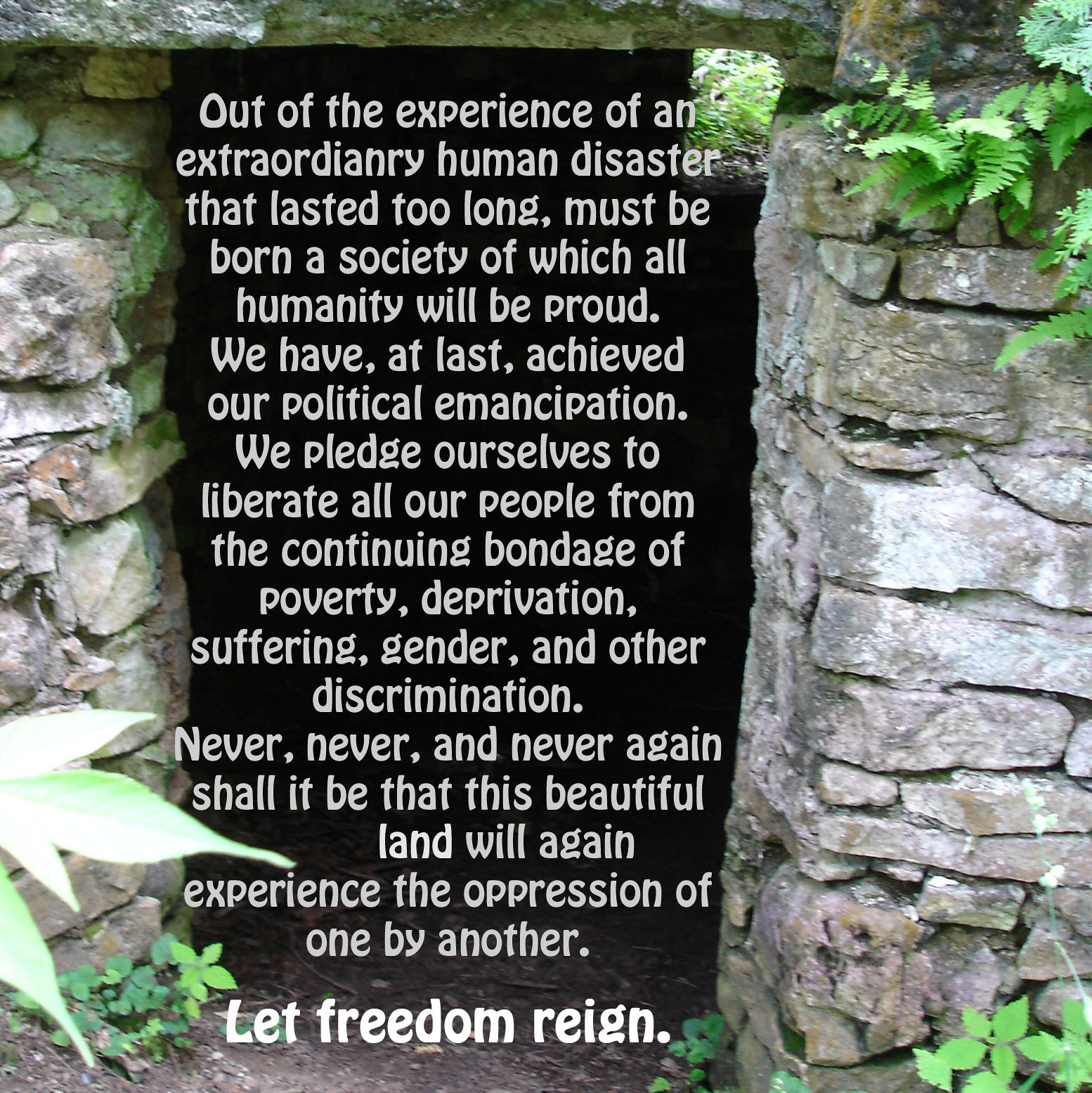The image showcases the entrance to an ancient cavern-like structure framed by rugged stone walls built from hand-hewn bricks. The entrance, shrouded in darkness, prominently features a compelling inscription in white text against the black background of the cavern's opening. The inscription reads, "Out of the experience of an extraordinary human disaster that lasted too long must be born a society of which all humanity will be proud. We have at last achieved our political emancipation. We pledge ourselves to liberate all of our people from the continuing bondage of poverty, deprivation, suffering, gender, and other discrimination. Never, never, and never again shall it be that this beautiful land will again experience the oppression of one by another." At the bottom, it concludes with the powerful statement, "Let freedom reign." Flanking the entrance are stacks of stones in shades of gray and white, sporadically touched by green shadows. Vegetation, including ferns and large green leaves, grows around and through parts of the stone structure, reflecting white light and adding to the ancient, yet vibrant, natural setting.